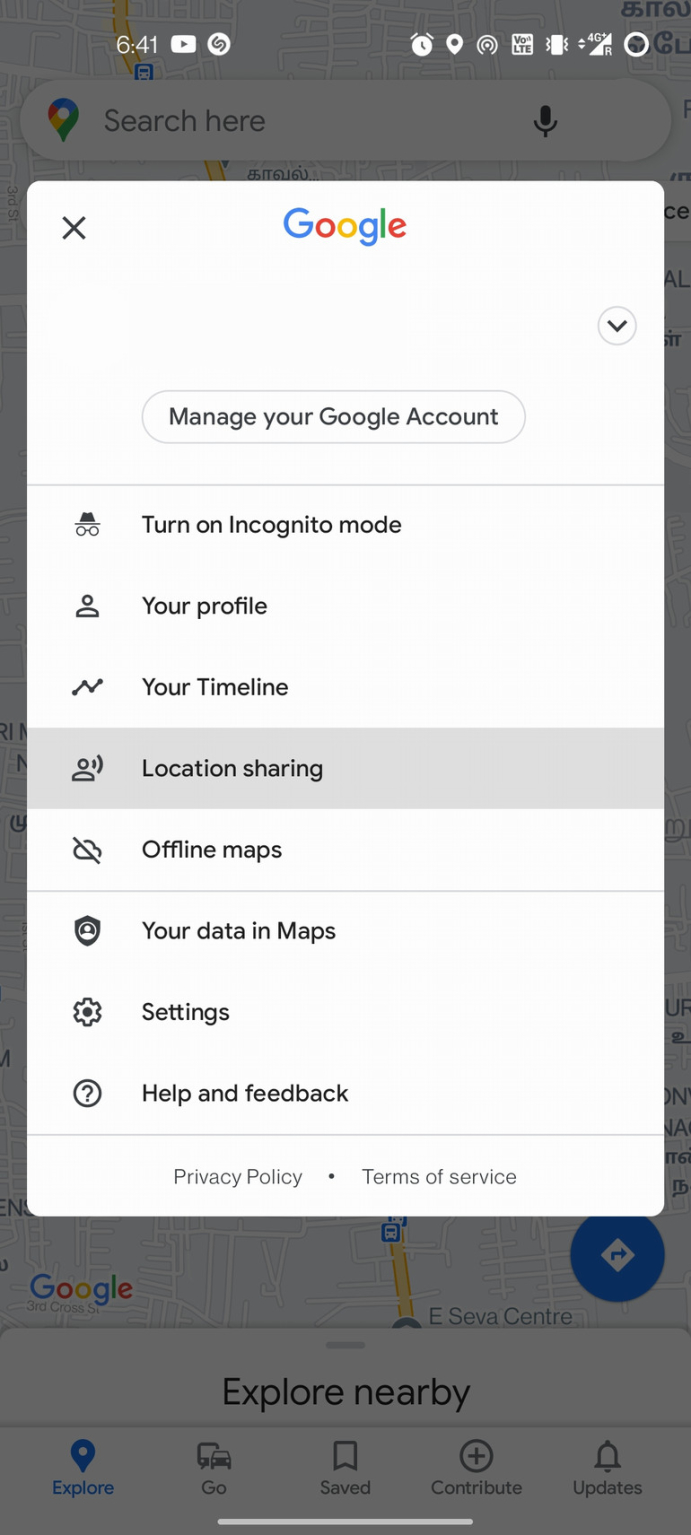The image depicts a smartphone screen displaying a layered view of Google Maps and a pop-up menu. 

At the very top, the screen shows the usual status indicators: the number "641" is visible, accompanied by a gray arrow inside a white box, a white circle with a gray squiggly line, a phone icon, a location icon, a volume icon, and a battery icon. The device is connected to a "4G-R" network.

The main background is the Google Maps interface. At the top of the Google Maps page, the search bar is prominent, displaying the placeholder text "search here" with a location marker icon on the left, colored in Google’s signature colors. On the right of the search bar is a black microphone icon. 

A white pop-up menu titled “Google” overlays the Google Maps page. At the top of this pop-up, the Google logo is displayed in its full-color glory. Below the title, it says "Manage your Google Account." The menu lists several options, each accompanied by a small black icon for quick identification: 
- Turn on Incognito mode with the incognito icon,
- Your Profile,
- Your Timeline,
- Location Sharing (shaded in gray from left to right),
- Offline Maps,
- Your Data in Maps,
- Settings,
- Help and Feedback.

At the bottom of the pop-up, links to the "Privacy Policy" and "Terms of Service" are provided. An 'X' icon in the upper left corner of the pop-up allows users to close the menu and return to the Google Maps screen.

In the muted background, obscured by the pop-up, the Google Maps interface continues. It includes an "Explore nearby" feature, with Google’s logo on the left and a blue circle for directions. At the very bottom of the screen, a navigation bar offers further options: "Explore" (highlighted in blue with a corresponding location marker), "Go" (with icons for a car and bus), "Saved" (marked with a save icon), "Contribute" (featuring a circle with a plus sign), and "Updates" (indicated by a bell icon), all in black text.